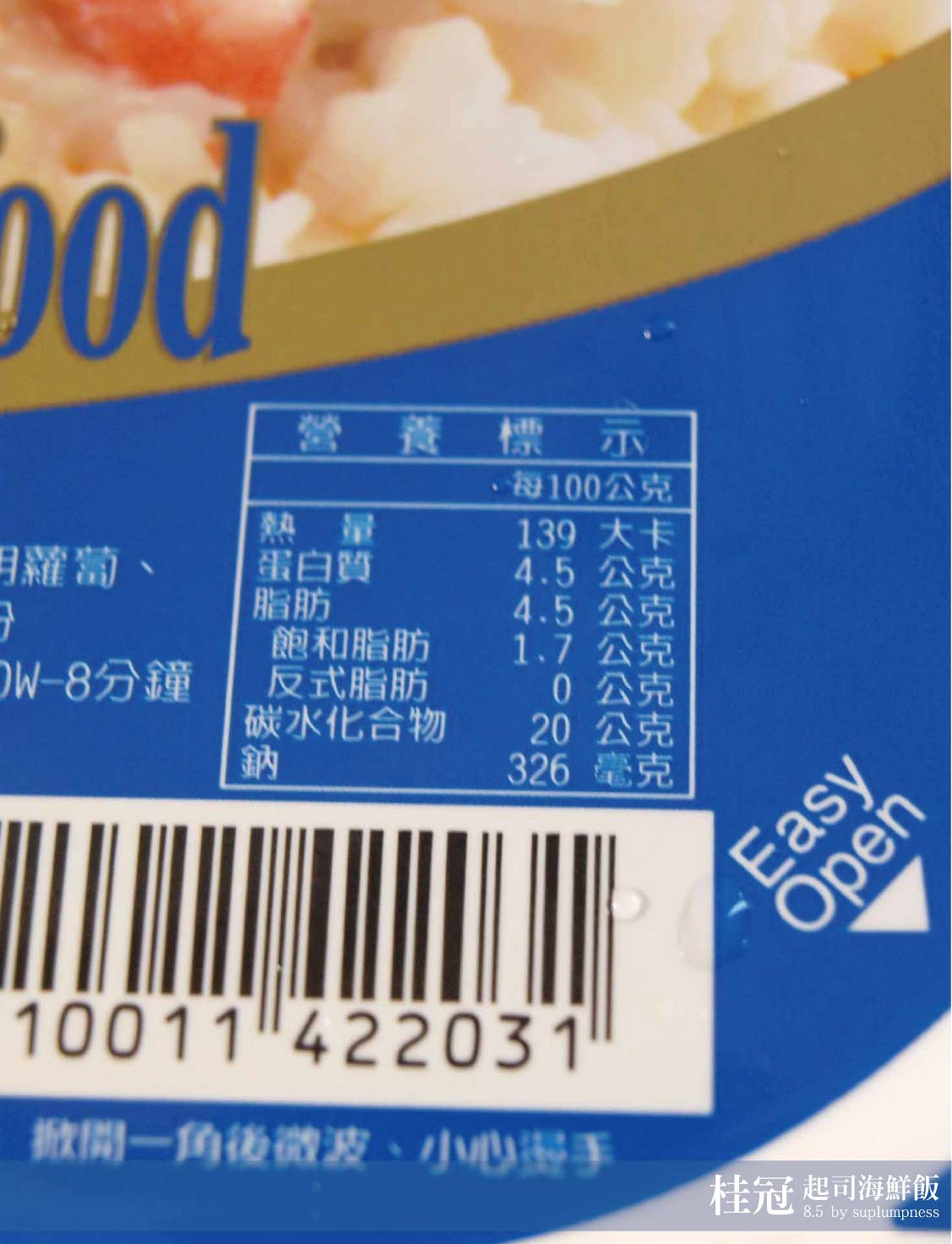The image captures a close-up of a blue food package, predominantly featuring nutritional information displayed in Japanese. The majority of the package's text is non-English, though notable English phrases including "Easy Open" can be seen in the bottom right corner. This English phrase is accompanied by a small arrow indicating where to open the box. Adding detail to the background, a gold band rests just above the blue section, which holds both the nutritional label and a near-complete view of the UPC barcode (10011422031). Although speculated to be a package for items like popcorn, ramen, or noodles, the actual food item remains unclear due to the limited visible imagery and obstructed packaging.